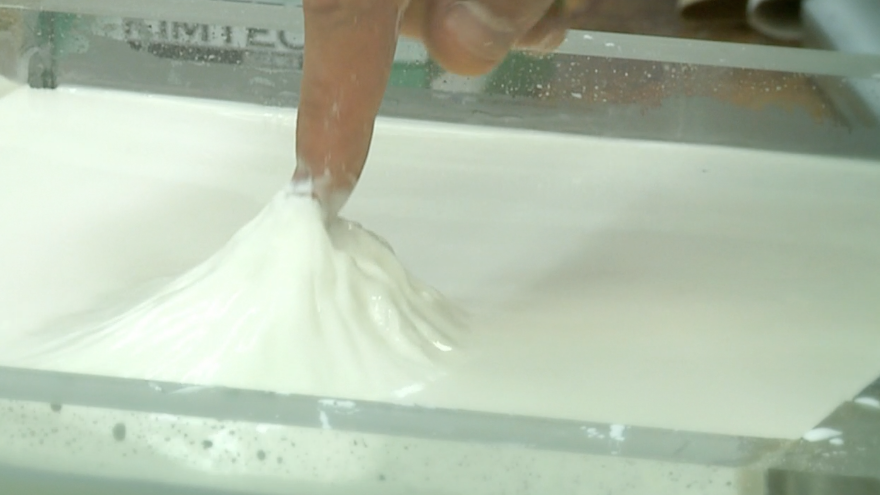The image depicts a laboratory-like setting where a white, pudding-like substance is contained within a thick, transparent, glass dish. The dish, featuring substantial walls about a quarter to half an inch thick, holds the smooth, glossy white substance, which resembles glue or yogurt in texture. A human finger is shown dipping into the material and lifting it, creating a noticeable mound that clings to the finger, highlighting the substance's high viscosity and sticky nature. The surface of the white liquid around the finger remains exceptionally smooth, emphasizing the contrast between the undisturbed and manipulated areas of the substance.